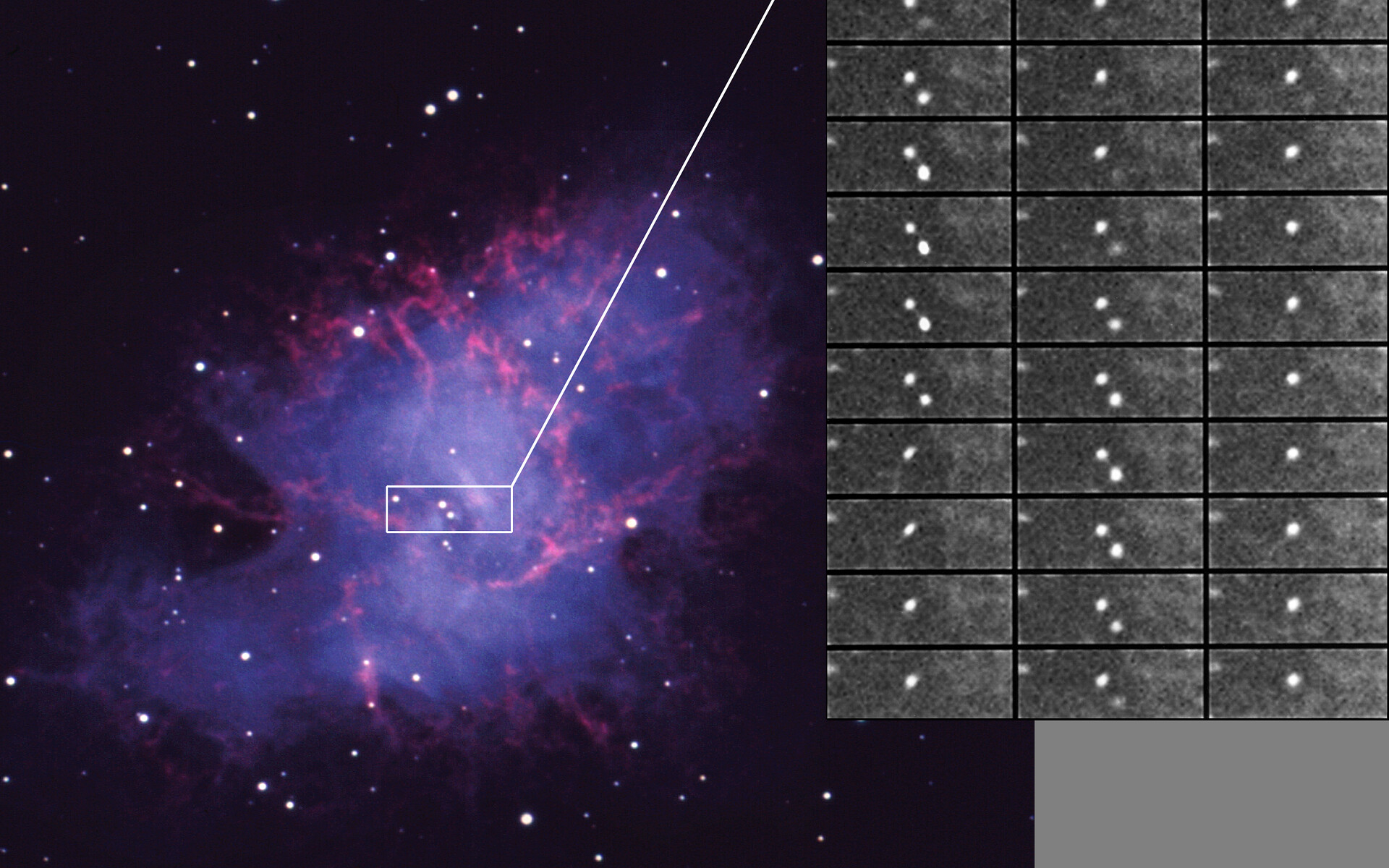This image appears to depict a celestial scene, likely a nebula in outer space, characterized by a purplish-pink, smoky area occupying the central portion of the frame. This nebula is set against the vast blackness of space sprinkled with numerous white and yellow stars. To the left, the nebula displays bright white highlights within its colorful expanse. 

On the bottom right, the image features a distinctive series of three vertical rows of gray rectangles, each containing one or two white dots, resembling a grid or diagram. Additionally, there is a diagonal white line extending from this grid towards the nebula, ending at a small white box that encloses three of the stars, seemingly highlighting them for emphasis or further study. The contrast between the vivid nebula and the structured gray grid provides an intriguing juxtaposition, suggesting a blend of natural celestial beauty and analytical observation.